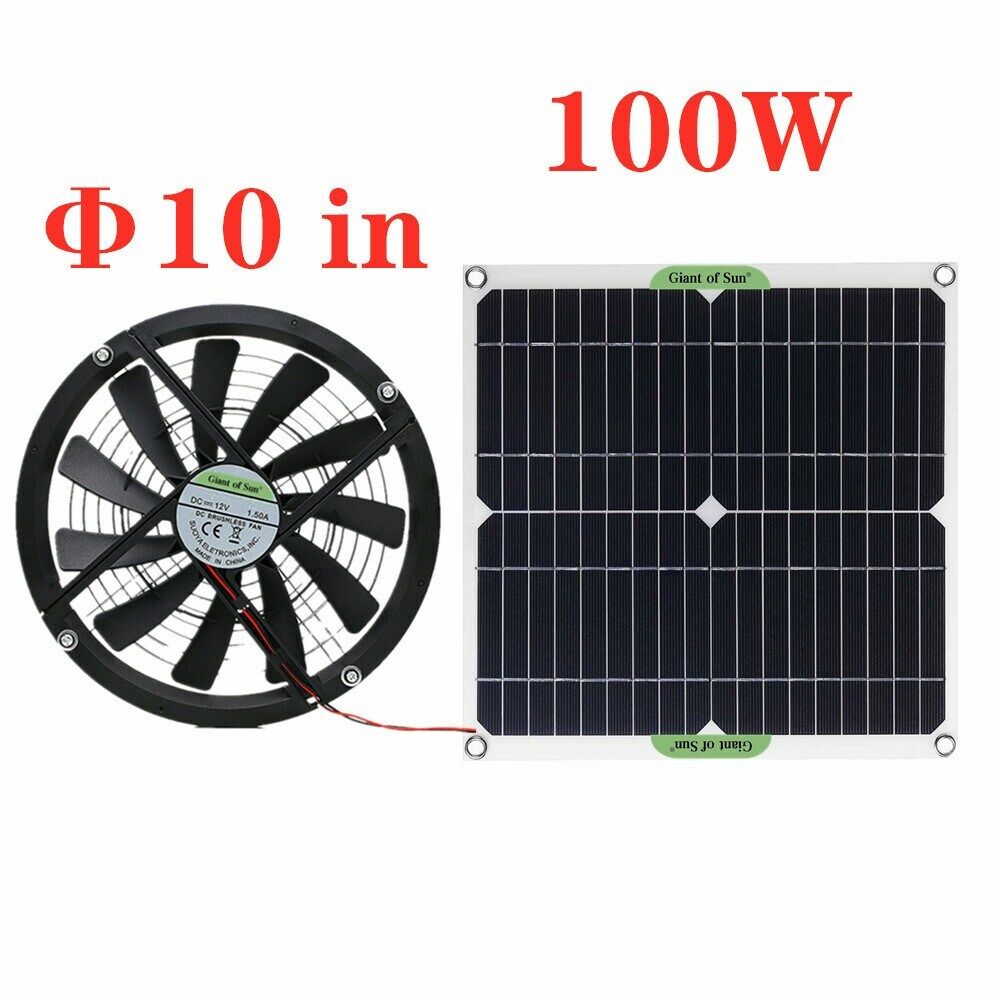The image depicts a detailed illustration of a hybrid fan and solar panel device. On the left side, there is a circular fan with multiple curved, rectangular blades that are black in color. These blades are protected by a metal grille composed of tiny iron rods and are mounted on a larger black circular base with four screws. At the center of this circular base, there is some writing, although it is not clearly legible. 

A prominent red wire extends from the center of the fan and connects to a square solar panel on the right side of the image. The solar panel, which has a silver frame, features black solar cells arranged in horizontal strips with silver linings between them. There is a small diamond-shaped detail and circular holes located at each corner of the panel, suggesting mounting points. 

Text appears above both the fan and the solar panel. "10 inch" is written above the fan, indicating its size, while "100 W" is written above the solar panel, signifying its power rating. The background of the image is black, providing a stark contrast to the outlined objects.